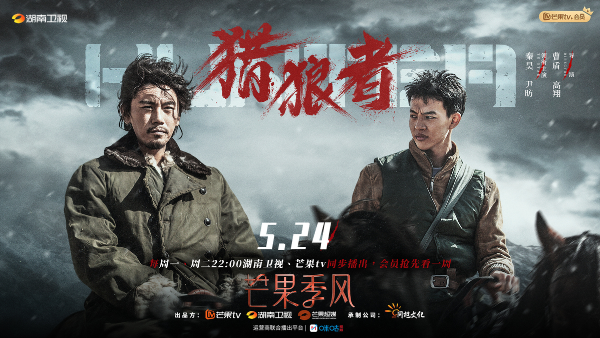The image appears to be a promotional poster, possibly for a Chinese action movie or video game, set to release on May 24th (5.24). It has an animated yet realistic look, with text in an Asian language, likely Chinese. The text includes bold red characters at the top and smaller ones in white, red, and orange at the bottom. The scene features two Asian men riding horses against a stormy, snowy background, their hair dramatically blowing in the wind. The man on the left has wild, semi-short hair and is dressed in an army green coat, while the man on the right sports shorter hair and wears a black vest over a brown coat. The man on the right appears to be staring at the other with a disgusted expression, adding a sense of tension to the image.